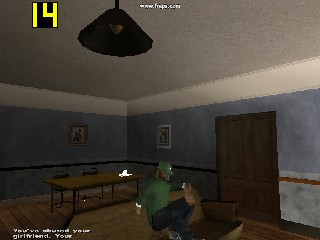This computer-generated image depicts a detailed game scene set in a room characterized by its distinct architectural and furnishing elements. The gray ceiling features a prominently hung black light fixture in the foreground. White trim elegantly outlines the ceiling, complementing the blue walls beneath it, which are accentuated by a chair rail dividing the upper and lower sections.

On the right-hand side of the scene, a white door stands slightly below the chair rail, creating a sense of depth and perspective. To the left of the door, the lower half of the wall continues with blue paneling leading to the back wall, maintaining the room's consistent color scheme.

In the foreground, a long wooden table dominates the visual space, positioned on a rich, wooden floor that adds warmth to the setting. Seated on the floor in front of the table is a character dressed casually in a green baseball cap, a matching green shirt, and black pants, adding a human element to the otherwise static environment. The overall composition effectively combines these elements to create an immersive and engaging game scene.